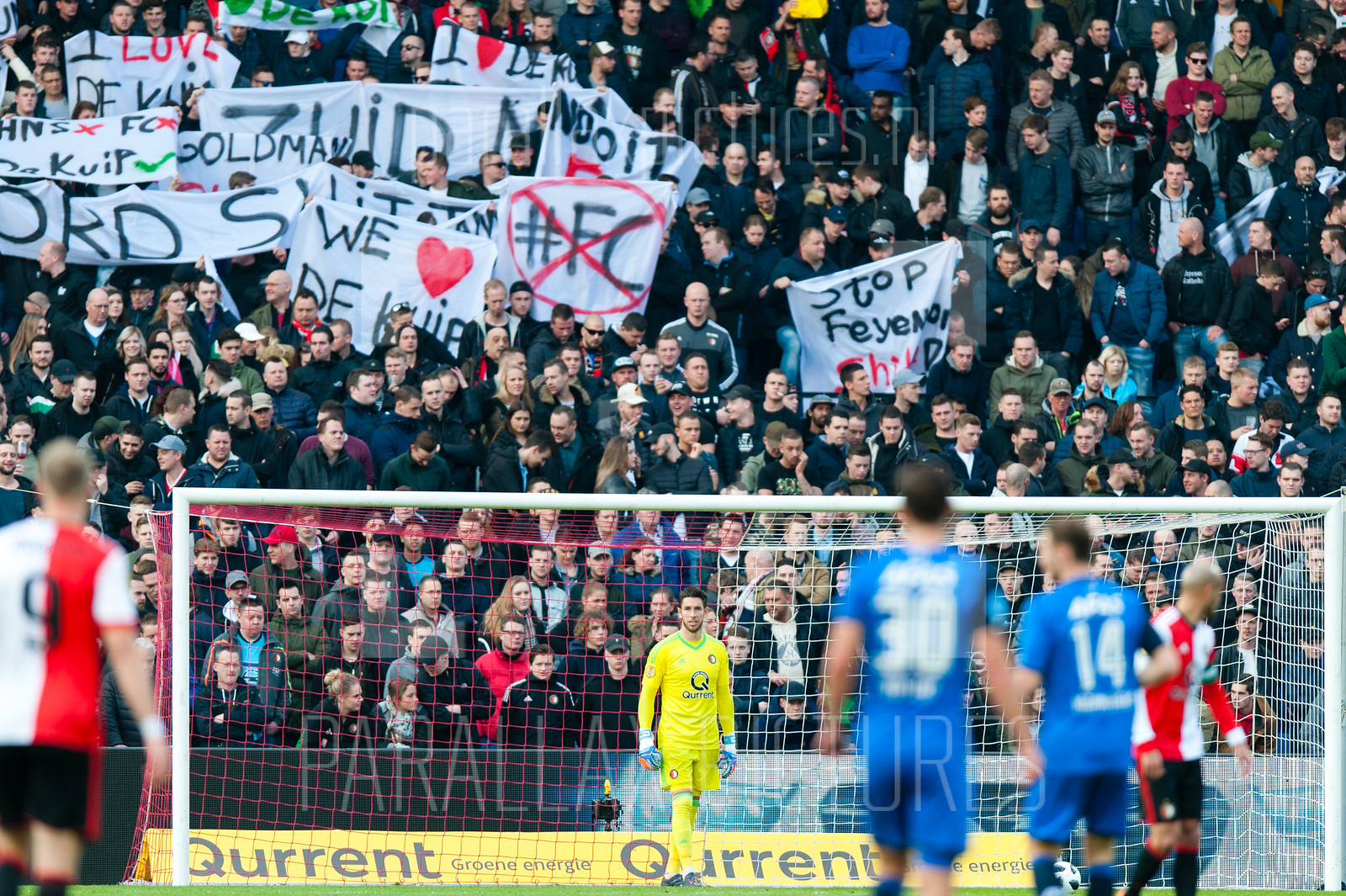This striking photograph captures a vibrant moment from a soccer match, taken from pitch level, facing towards the end zone. In the foreground, the entirety of the white goalpost with netting is visible, guarded by a goalkeeper clad in a prominent yellow uniform. Two players in blue and white jerseys face the goalkeeper, their backs turned to the camera. Additionally, two other players, possibly officials, wearing red and white vertically striped jerseys and black shorts, are present further out, although their faces are blurred.

Prominent in this image is the massive crowd of spectators that fills nearly the entire background. This enthusiastic audience is standing, many wearing dark coats and jackets, and they are fully engaged with the on-field action. Several attendees are holding handmade signs with various messages, including ones that say "Stop Fahrener," a hashtag with "FC" crossed out in red, and another sign which faintly reads "Weheartdkup" or similar. One of the signs appears to bear the word "Goldman."

Adding to the scene's vibrancy, a bright yellow barrier labeled "Corinth" (spelled Q-U-R-R-E-N-T) stretches across part of the viewing area, adding to the graphic elements that frame this dynamic shot.